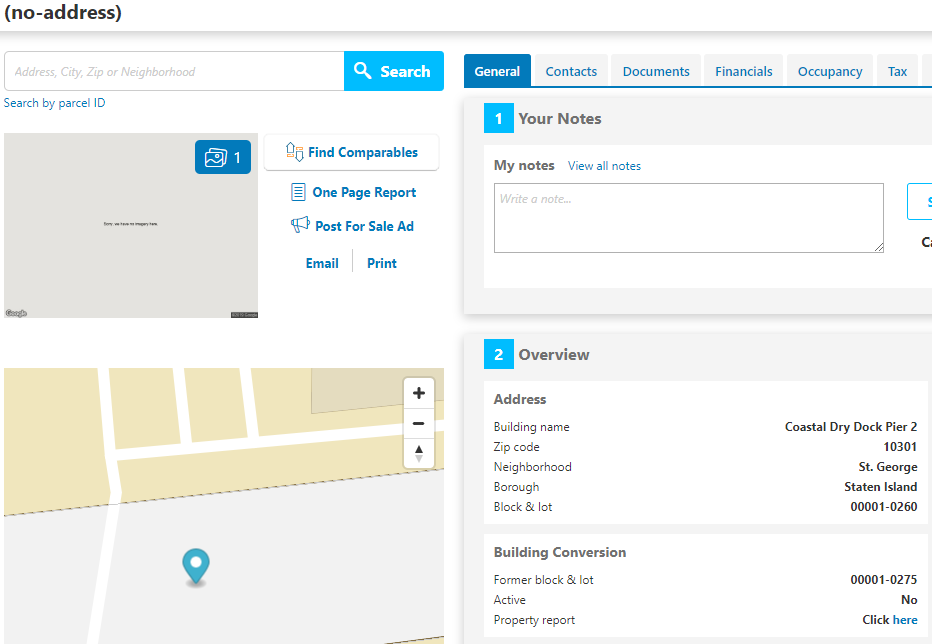The interface features a structured layout designed for property search and management. 

On the top left, there is a section for the user's address entry, including a field for the address and ZIP code. Adjacent to this, a prominent blue button labeled "Search" facilitates quick searches. Below this, users have the option to search by Personal ID.

In the subsequent section, a grey box is displayed, showing a singular image in the top right corner. Next to the image, a clickable blue button labeled "Find Comparables" is provided. Additional actionable buttons include:
- "One Page Report"
- "Post for Sale Ad"
- Options for email and print actions

Continuing down, there's a Google map with a marked blue pin. Above the map, a horizontal dotted line guides the eye across the segment. Zoom controls (+ and -) are situated at the top right of the map section.

The top right above the search bar lies the navigation tabs, which include:
- General
- Contact
- Document
- Financial
- Occupancy
- Tax

The "General" tab is currently active, indicated by its blue color.

Directly underneath, there is a numbered blue box labeled "1" with "Your Notes" next to it. There is an option for users to add or view all notes, enabling note management.

Following, another box is labeled "2" with an adjacent blue button labeled "Overview". This includes detailed property information such as:
- Address: Coastal Drag Dock, Pier 2
- ZIP Code: 10301
- Neighborhood: St. George
- Borough: Staten Island

Additionally, details of building conversion to the status "000010275 active" are provided, though marked as "no". A clickable "Property Report" link is also available, highlighted in blue for ease of access.